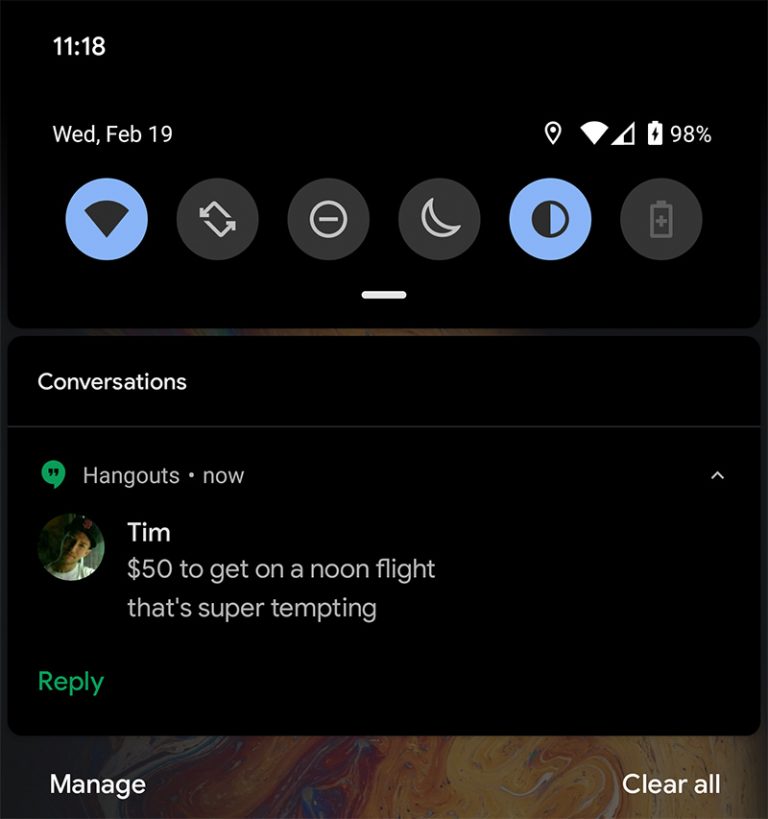In the image, a close-up screenshot of a phone's display is captured, set against a predominantly black background. In the top left corner, bold white text reads "11:18," and just below it, "Wed, Feb 19," indicating a timestamp. Adjacent to the right, there is a series of icons including a location indicator resembling a windshield, a Wi-Fi signal icon, and a battery icon displaying "98%."

Beneath this section, a row of six circular icons is visible:
1. A light blue icon with a black windshield symbol.
2. A grey icon featuring two arrows forming a rectangular loop.
3. A white circle with a horizontal line across the center.
4. A crescent moon icon.
5. A yin and yang symbol where one half is light blue and the other is black.
6. A light grey icon depicting a battery with a plus sign inside.

Further down, another section labeled "Conversations" in small white font appears. Under this heading, a grey bar separates the section titled "Hangouts." Here, a green chat bubble icon precedes text indicating a new message, with "now" noted beside a dot.

Below, the message interface shows a man named Tim—depicted as a Caucasian male with a ball cap featuring a red insignia. His message reads, "$50 to get on a noon flight, that's super tempting." To the left of his message are options to "Reply" in green and "Manage" in white text, while "Clear all" is displayed to the right.

The phone's wallpaper in the background showcases a vibrant representation of Jupiter's swirling layers in hues of orange, yellow, blue, and white.